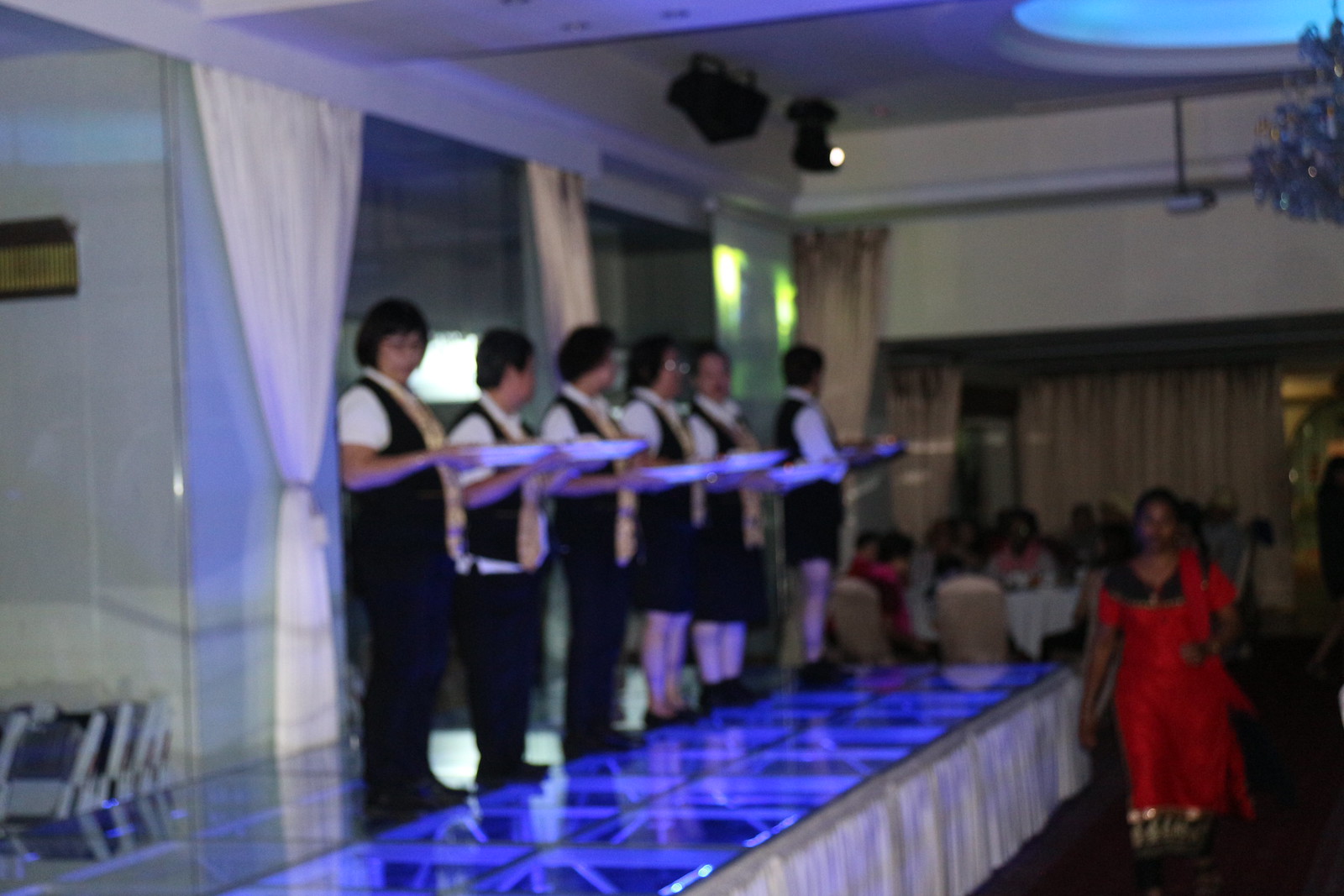This slightly blurry and somewhat dark image captures an indoor dining venue, possibly hosting a celebratory catered event, such as a reception or special dinner. In the foreground, six individuals, uniformly dressed in white short-sleeved shirts beneath black vests and either black pants or skirts, are lined up on a glass-covered stage. Each server holds a white platter, which glows faintly under the stage's blacklight illumination. The stage itself is elevated on visible metal scaffolding and is illuminated with a blue hue from below. Behind the servers, white curtains hang and two black devices, likely lights or projectors, are mounted above. In the background, diners are seated at tables, contributing to the lively atmosphere. To the right of the stage, a woman in a red sari-like outfit and dark hair walks towards the camera, her elegant attire enhancing the sense of occasion. The image depicts a scene of preparation and service, suggesting that the waitstaff is getting ready to serve the attending guests at this undoubtedly special event.